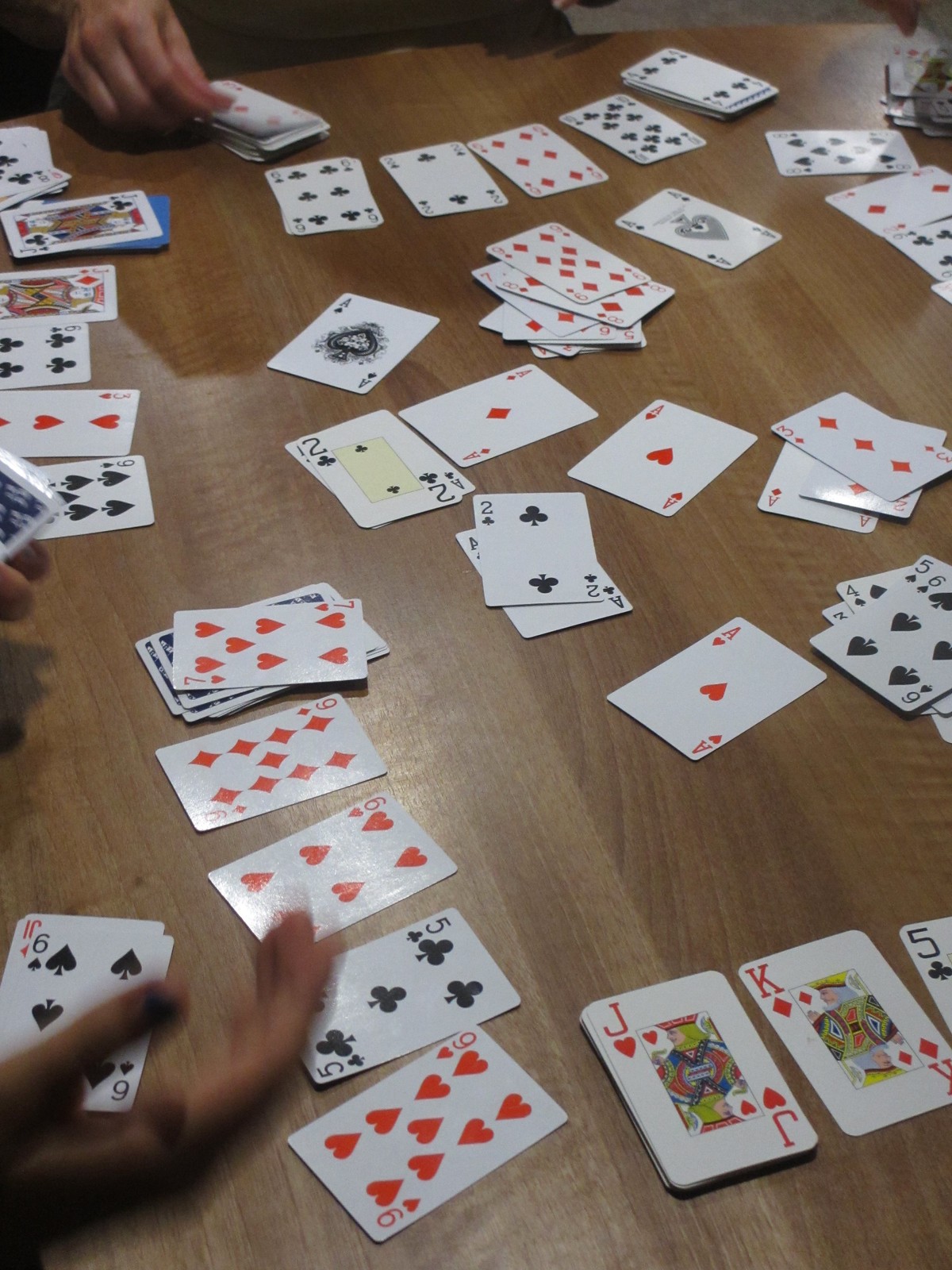In this detailed image, a wooden brown table takes center stage. On the table, there is a deck of cards spread out haphazardly, with some cards stacked neatly while others are scattered messily. The image captures the intensity of a card game in progress, as evidenced by multiple pairs of hands actively engaging with the cards. One player's hand is shown picking a card from one of the stacks, indicating a moment of decision in the game. The scene exudes a lively and competitive atmosphere, with the players deeply engrossed in their game.